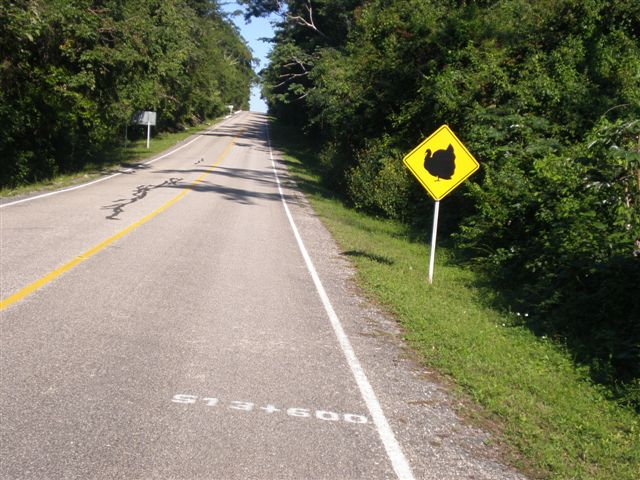A rural two-way street stretches before us, defined by a yellow dividing line and bordered by white lines on each side. The asphalt surface bears white markings reading "S13 + 600." Lush green grass flanks the road, with tall, bushy trees providing a verdant backdrop. On the right side of the road stands a yellow, diamond-shaped street sign featuring a silhouette of a turkey, indicating a cautionary warning for potential turkey crossings. Above, the sky is a clear blue, reflecting the bright and sunny weather conditions.